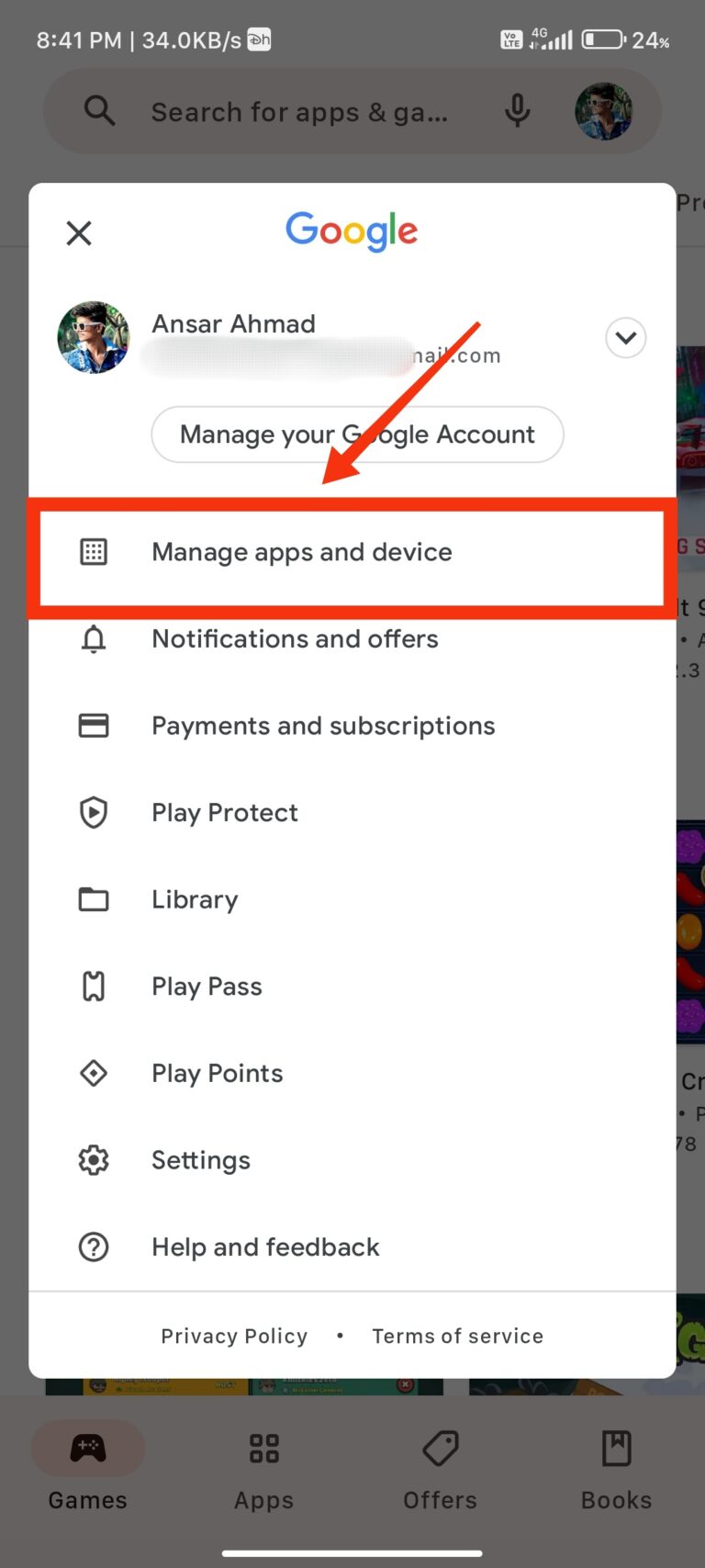A detailed screenshot depicts a user interface from a smartphone with a gray background. At the top left, the time is displayed in white text along with data transfer information "34.0 KB/s." On the top right, icons for battery, network reception, and other status indicators are visible. Directly beneath, a search bar is centrally positioned, featuring a black magnifying glass icon on the left, and the text "Search for apps & GA..." in black is centered inside. To the right of the search bar are a microphone icon and a profile icon.

Below the search bar, a large white rectangle hosts the rest of the interface. In the top left of this rectangle, a black "X" is displayed, while the word "Google," colored in the signature Google colors, is centered at the top. Just a few lines down, the profile icon and the name "ANSAR AHMAD" are to the left, with grayed-out text beneath the name. To the right of the profile line, a downward arrow is present. Immediately beneath is a centered button reading "Manage your Google Account" with gray text on a white button.

Further down the list, several menu items appear in gray, each accompanied by a corresponding icon on the left: "Manage apps & device," which is notably outlined with a thick red border and has an arrow pointing to the word "apps" starting from the upper-right corner, "Notifications & offers," "Payments & subscriptions," "Play Protect," "Library," "Play Pass," "Play Points," "Settings," and "Help & feedback."

Finally, at the bottom of the screen, there are two options: "Privacy Policy" on the left and "Terms of Service" on the right.